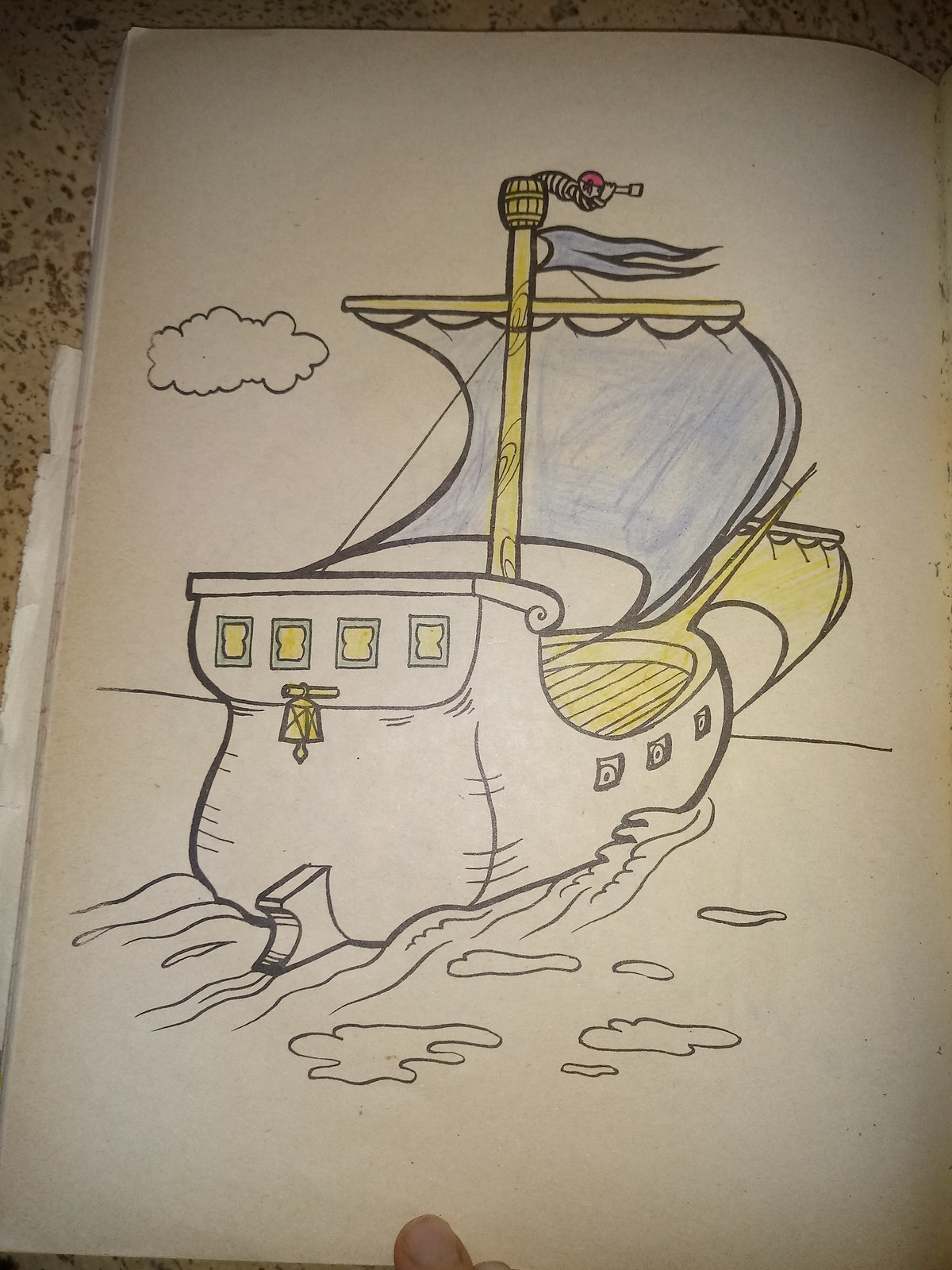This is a photograph of a detailed drawing of a pirate ship, created on a piece of sketchbook paper, which is slightly faded and appears old. The drawing is placed on a beige and brown quartz or Corian counter, with the top left and top of the image revealing a marble surface with brownish spots. The pirate ship is depicted sailing away from the viewer, diagonally towards the top right corner of the page. The ship's deck and various wooden parts are primarily colored yellow, including the mast, crow's nest at the very top, and another sail at the front. The main sail and flag are blue, gently blowing in the wind. At the stern of the ship, there are four yellow windows in a row, and below them is a post with a yellow lantern hanging. On the bow, a very pointy structure, resembling a unicorn horn, juts out prominently. A man with a black and white striped shirt and a red bandana stands in the crow's nest, peering through a telescope. The water beneath the ship remains uncolored, and the trails of water suggest the ship is in motion. A solitary cloud is shown in the top left corner of the image. At the bottom middle of the page, a finger holds the sketchbook open, and a sliver of the next page is visible at the top right.